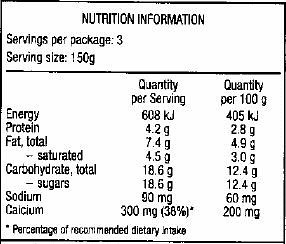This image depicts a detailed nutritional information chart typically found on food packaging. The chart is presented in black print on a white background and is enclosed in a black squarish outline. At the top, it prominently states "Nutrition Information". Below this, it indicates that there are three servings per package, with each serving size being 150 grams.

A black horizontal line separates the header from the nutritional details. The chart is organized into three columns, listing various nutrients and their respective quantities both per serving and per 100 grams. The first item is energy, noted as 608 KJ per serving and 405 KJ per 100 grams. Following energy, the chart lists protein as 4.2 grams per serving and 2.8 grams per 100 grams, fat total as 7.4 grams per serving and 4.9 grams per 100 grams, saturated fat as 4.9 grams per serving and 3.0 grams per 100 grams, carbohydrates total as 18.6 grams per serving and 12.4 grams per 100 grams, sugars as 18.6 grams per serving and 12.4 grams per 100 grams, sodium as 90 mg per serving and 60 mg per 100 grams, and calcium as 300 mg (38% of recommended dietary intake) per serving and 200 mg per 100 grams. 

At the very bottom of the chart, a black asterisk precedes the note about the "percentage of recommended dietary intake." Notably, the chart does not specify the type of food or list any ingredients. The grainy quality of the image suggests it might be a photograph rather than a digital rendering.